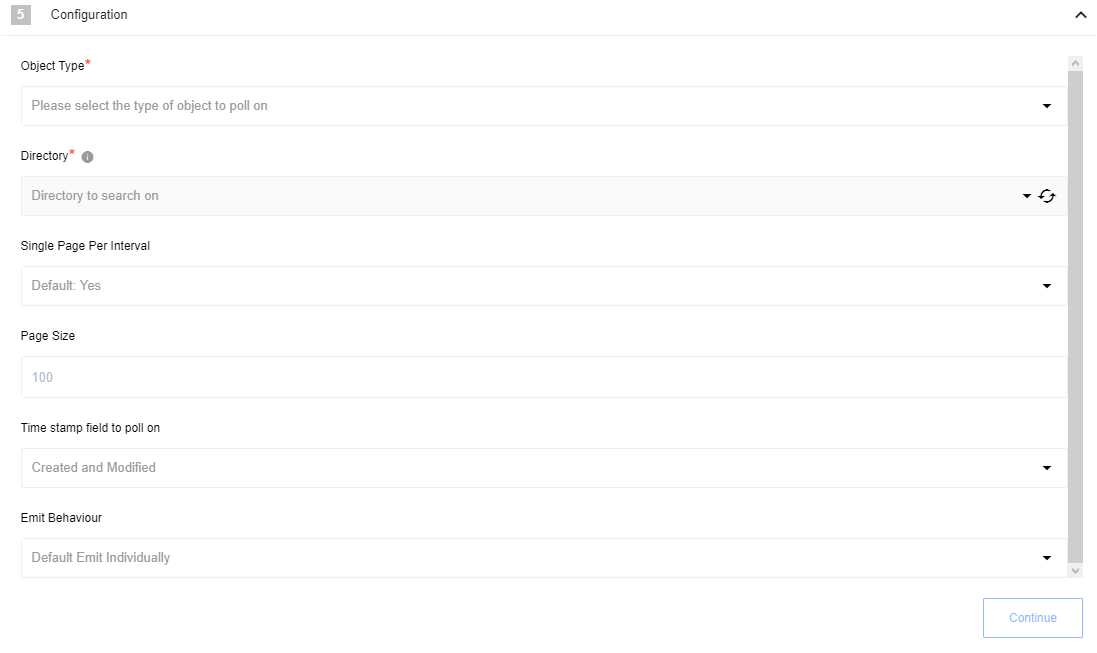The image depicts a detailed user interface screen, primarily featuring a configuration panel located in the top-left corner. This panel is labeled "Configuration" and has an "Object Type" field set to "Star." Users are prompted to select the object type from a drop-down menu, which defaults to "Module."

Below this, there is a section labeled "Directory," featuring another dropdown for "Directory Search," allowing users to explore directory options. Further down is an option for a "Single Page Printable," which is toggled to 'Yes.' The page height is specified as 100.

Two timestamp fields are present, labeled "Create" and "Modify," indicating the types of timestamps to be pulled. Another section displays "Emit Behavior," which is set to the default "Emit Individually."

A prominent blue square button labeled "Continue" is situated in the interface, ready to be clicked to proceed. Adjacent to this button, towards the right, a gray bar is visible, which contains various line and square icons along with different input fields, text boxes, and drop-down menus. This section is also equipped with up and down arrows for navigating options.

The overall background of the interface is white, providing a clean and organized look to the layout.